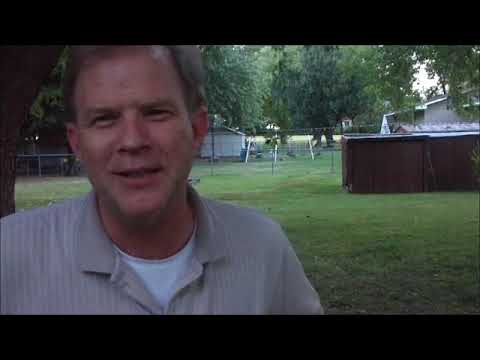The image depicts a middle-aged white man with slightly graying brown hair, wearing a gray striped collared shirt over a white undershirt. He is standing outside in a grassy backyard. He appears to be smiling faintly or possibly mid-conversation with someone off-camera, positioned close-up and to the left portion of the image. 

Behind him, the background features a residential setting including an above-ground pool with a brown exterior. To the right stands a long wooden shed adjacent to a chain-link fence. Beyond the fence, there is another yard containing a white shed, a variety of large green-leaved trees, and a house with gray walls and white trim. Additional elements in the backdrop include a clothesline, a brown tree trunk, and scattered patches of dirt. The photograph is taken during the daytime as evidenced by the light filtering through an opening in the trees. Both the top and bottom edges of the image have prominent black horizontal lines.